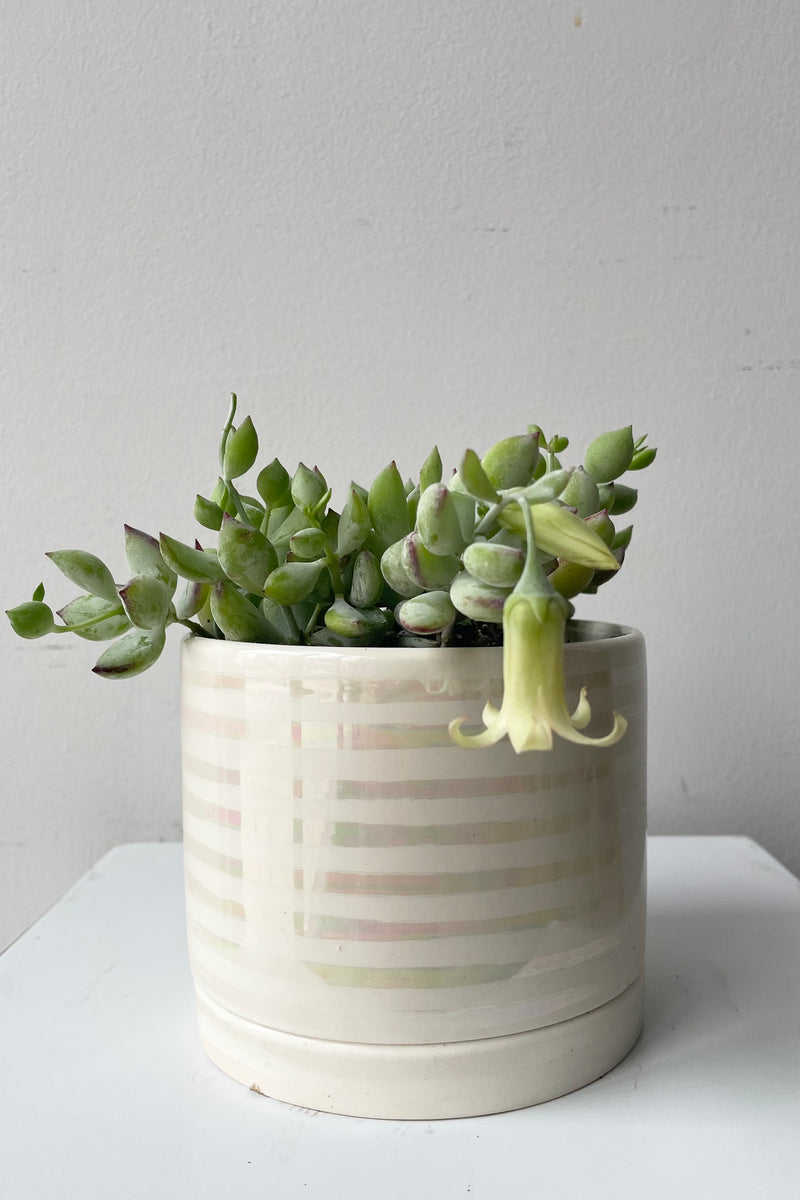This photograph features a cylindrical, white planter adorned with iridescent, horizontal grey stripes, housing a lush succulent. The succulent boasts a variety of plump, tapered, and rounded green leaves, creating a visually appealing mix of textures. Among the succulent leaves, a bell-shaped flower hangs over the edge of the pot, seemingly in bloom, while another flower angles at 45 degrees, yet to blossom. The scene is set against a light grey wall, with the planter resting on a square white table, and a water collection mechanism is visible at the base of the planter, emphasizing the indoor setting.